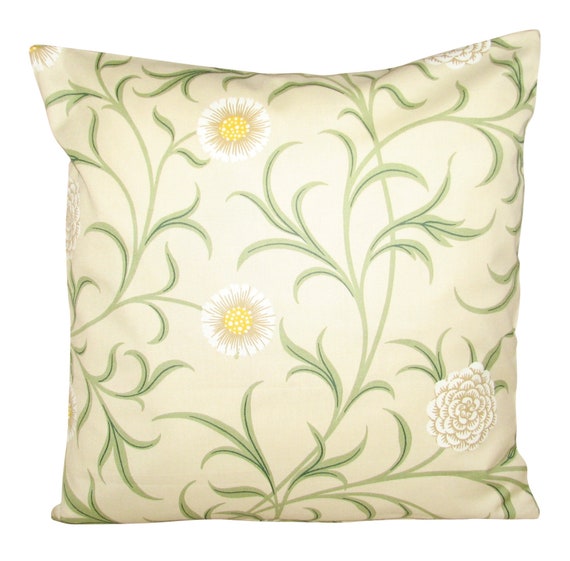This image depicts a plump, square-shaped pillow placed on a uniform white surface. The pillow, photographed from above, showcases an intricate design primarily consisting of plant motifs. The fabric of the pillow has a subtly shiny, satin-like texture, giving it a light, whitish beige or slightly greenish tan hue.

Adorning the pillow are light green, swerving branches with thin, dark green-lined leaves. Interspersed among the foliage are several flowers, including white chrysanthemums with dense white petals and dandelion-like flowers characterized by yellow centers and bristle-like white fringes. The dandelion-like flowers appear on the upper left, upper right, and lower right sections of the pillow, with some partially visible. This detailed, botanical-themed pattern gives the pillow a sophisticated and natural aesthetic.